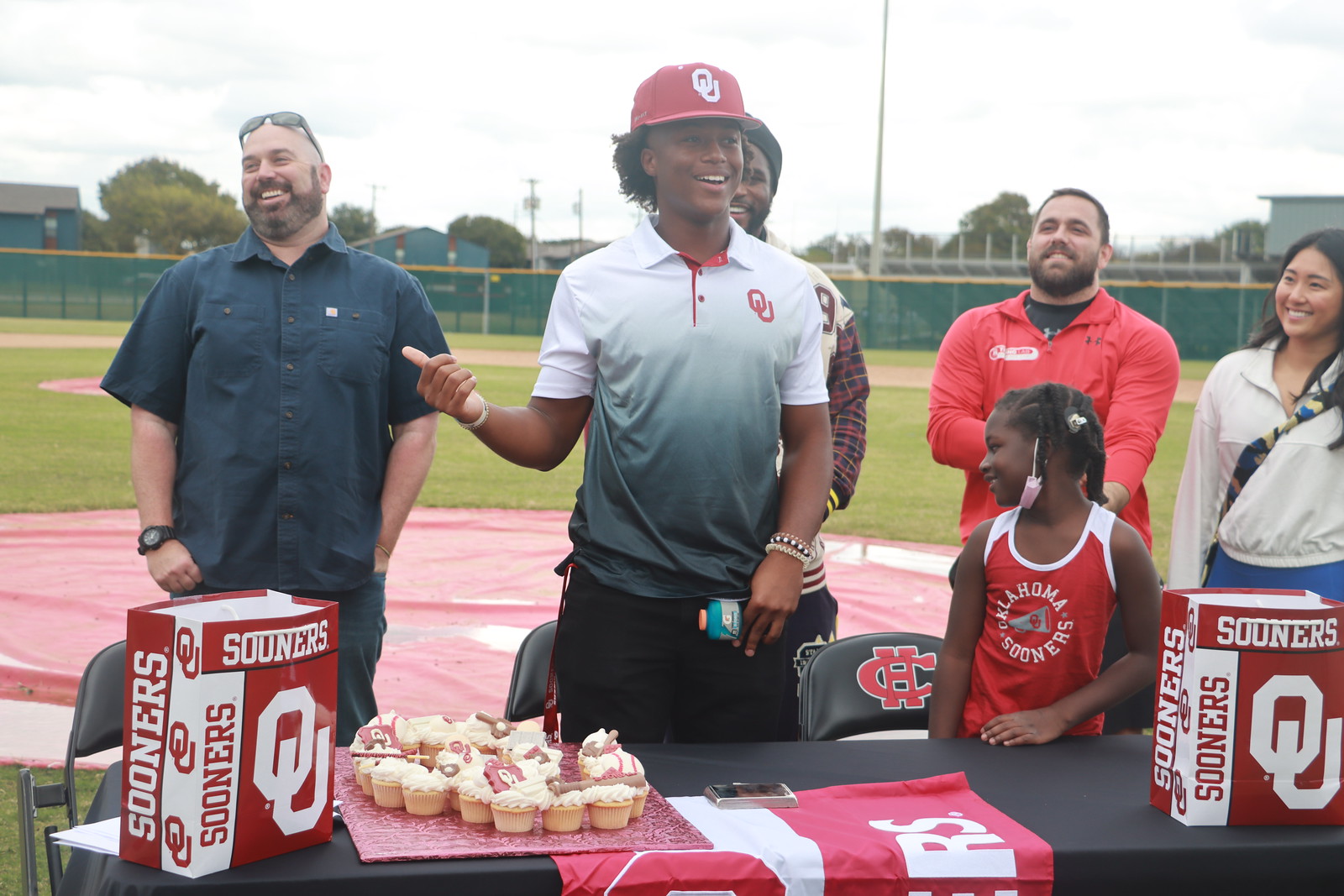The image captures a lively event taking place on a baseball field, presumably associated with the Oklahoma Sooners, given the prominent red and white logo and "Sooners" branding visible across various items. Central to the scene is a table covered with a black tablecloth, adorned with gift bags bearing the Oklahoma Sooners logo and a platter loaded with frosted cupcakes decorated with similar team insignias. Behind the table, a black chair with a "CH" logo adds an extra detail to the setup.

Numerous individuals are gathered around the table, highlighting the communal and festive atmosphere. An African American man, possibly in his late teens to late twenties, stands at the table. He sports a red Oklahoma Sooners baseball cap and a stylish polo shirt in white and gray with red accents and the OU logo. Next to him is a young African American girl in a red and white Oklahoma Sooners jersey. They are surrounded by other attendees, including an Asian female adult and an African American younger girl.

The backdrop features a black fence enclosing the field and a mostly cloudy sky, with daytime lighting casting soft shadows across the scene. Another notable figure is a man laughing heartily in the background, wearing a black short-sleeved button-up shirt and sunglasses perched on his head. The overall context suggests a spirited gathering or celebration, potentially in honor of the Oklahoma Sooners baseball team.